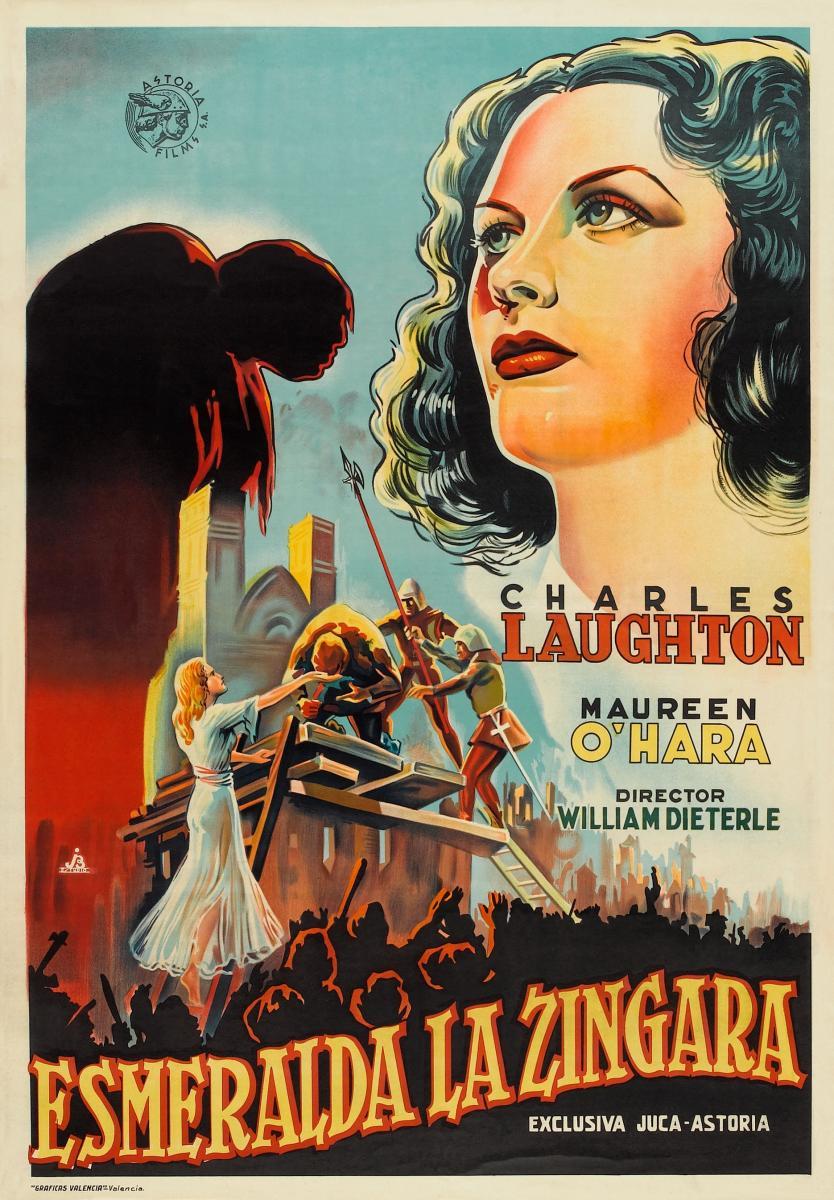The movie poster for "Esmeralda La Zingara" is a vertically oriented card with a cream border and a dark background that accentuates its vibrant elements. Along the bottom edge, the credits read "GRAFICRS Valencia Valencia," and prominently in yellow font with red trim, the title "Esmeralda La Zingara" stands out, followed by "Exclusiva JUCA - Astoria" in white. The poster features a dramatic scene where a barefoot woman with long blonde hair, wearing a translucent dress accented with a belt, is ascending a ladder. She appears to be aiding a man on a platform, potentially in the midst of an execution, while executioners loom at the top. The scene includes a large crowd below, creating a sense of urgency and tension. Additionally, the names "Charles Lawton," "Maureen O'Hara," and "director William DiTorelli" are listed to the right. The top right corner of the poster showcases the woman’s face, with long black hair and striking makeup, gazing to the left. The upper left corner features the icon logo of Astoria Films S.A., depicting a soldier-like figure reminiscent of Mercury. The backdrop includes elements like soldiers with bayonets and possibly the Notre Dame cathedral, indicating a potential Spanish version of "The Hunchback of Notre Dame."